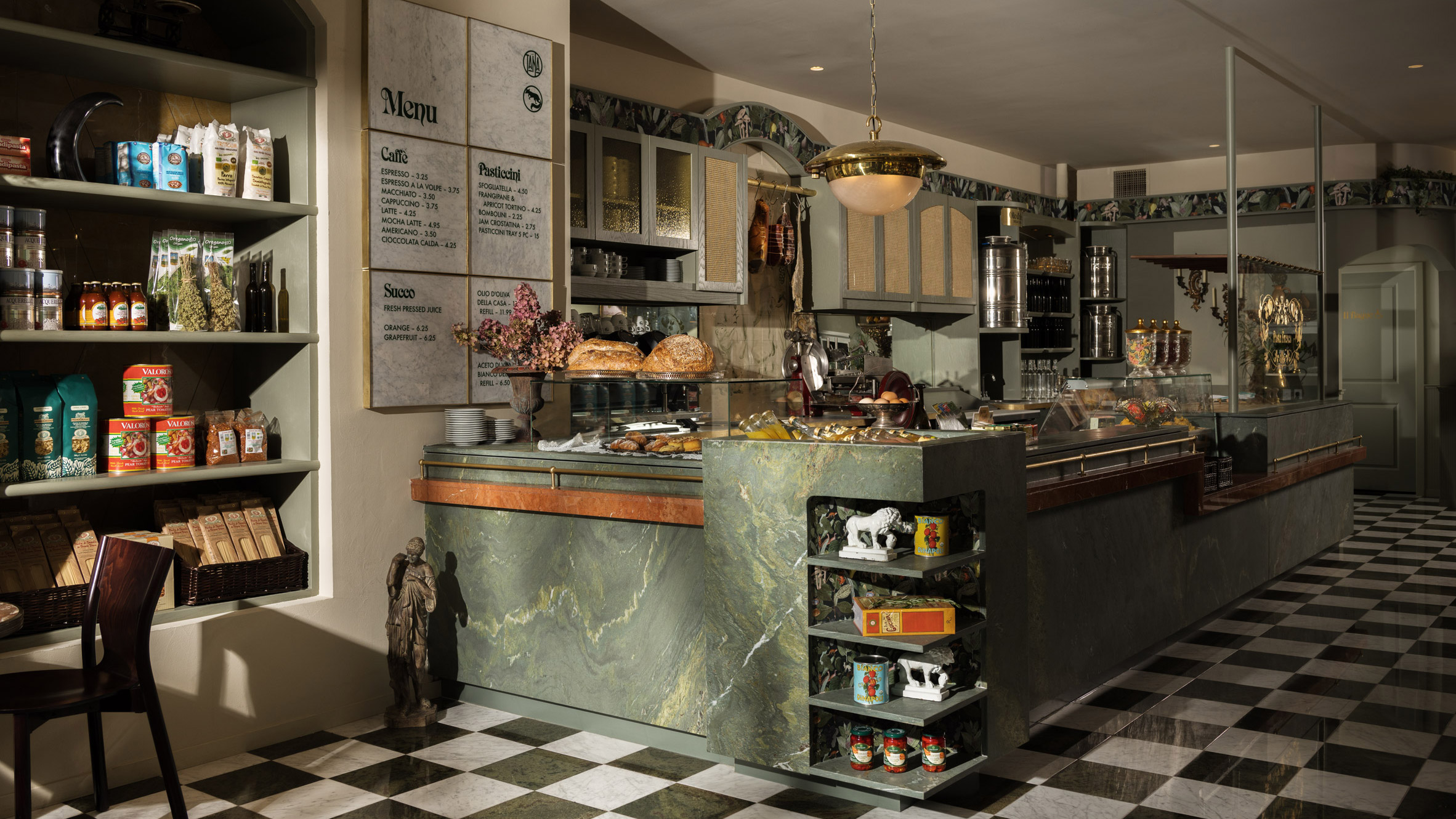The image captures the interior of what appears to be a small cafe or delicatessen. Centered in the photo is the serving counter, featuring a countertop made of green-gray marble. The floor is adorned with black and white checkered tiles, conveying a vintage ambiance. 

On the left side of the image, there are shelves displaying various products for sale, though the specifics of the items are unclear. Above these shelves hangs a chandelier with a metal cover, adding an element of sophistication to the space. 

To the right, there is a cabinet filled with what seem to be coffee products and other food items, emphasizing the shop's diverse offerings. The decor complements the antique style, featuring dark gray, black, and white colors. A menu is visible on the wall above the shelves, but the details are not legible. The photo lacks any human presence, putting full focus on the intricately designed interior of this charming shop.